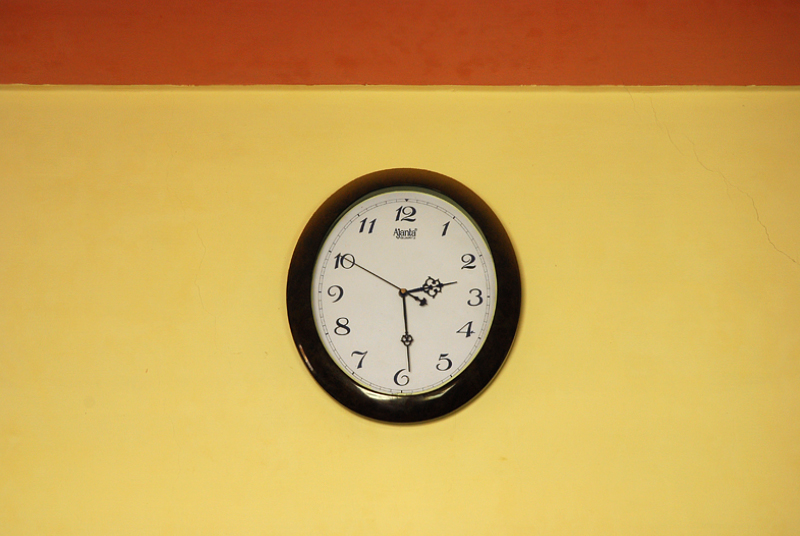In this vintage-style photograph, the image is oriented horizontally, providing an extended view of the scene. Dominating the composition is a round, vintage wall clock, which features a sleek black frame and a cream-colored face. The clock is adorned with bold, black numbers ranging from 12 to 11, circling its face. The black hour and minute hands point to 2:30, while the slender second hand is frozen at the 10-second mark. The clock is mounted against a vibrant banana yellow wall that contrasts sharply with the bright red ceiling above. Beneath the 12 o’clock mark, there appears to be a blurred brand name, possibly reading "Agamba" or "Ajamba," adding to the antique feel of the image. The photograph itself is of lower resolution, enhancing its vintage aesthetic and nostalgic appeal.